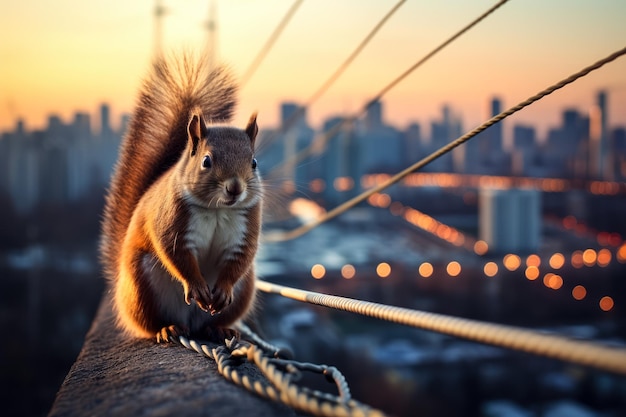In this photograph, a squirrel is positioned prominently on a concrete wall, seemingly perched above a misty, urban landscape. The squirrel, facing the camera, showcases its reddish-brown fur and distinctive white chest. Its tiny paws are held together in front of it, while its bushy tail arches gracefully over its back. To the right, five cable wires stretch diagonally across the frame, becoming progressively fainter as they extend upwards towards the top of the image. The bottom cable is the most in focus, while the others gradually blur into the backdrop of a vibrant sunset. The sky is a gradient of warm yellows and oranges, fading into deeper hues as it meets a soft, out-of-focus cityscape below. There is also a suggestion of water in the distant background. Additional cables can be seen running beneath the squirrel, partially embedded in the concrete wall. The overall composition juxtaposes the sharp, detailed image of the squirrel against the dreamy, indistinct surroundings, evoking a sense of serene solitude amidst urban life.